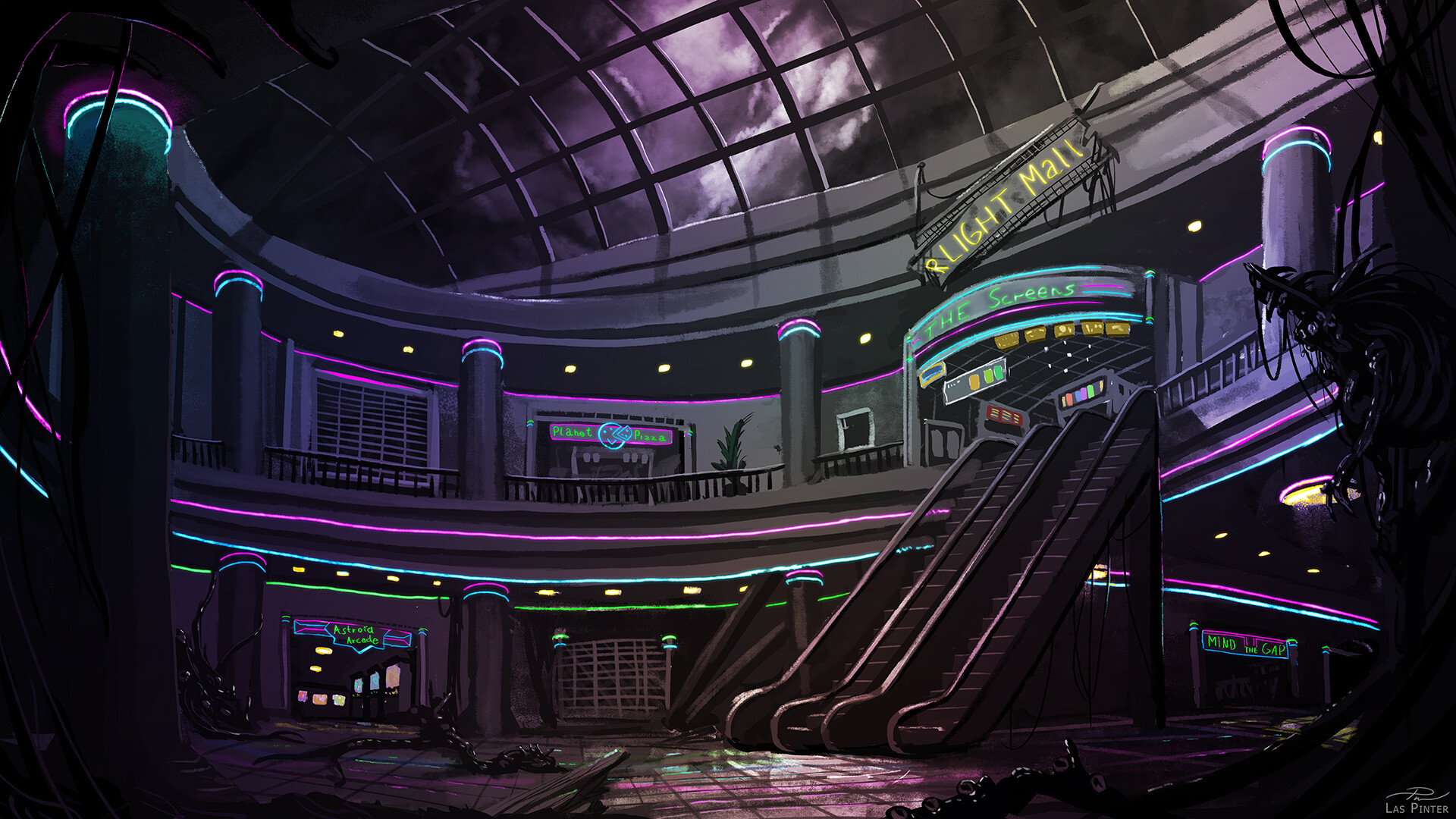This is a detailed, computer-generated image of a dark, artistic rendition of the central lobby area of a two-story, indoor mall. The overall color palette is predominantly charcoal gray with vivid blue and pink neon highlights. The image is set at night, as suggested by the purple sky and white clouds visible through the greenhouse-style, glass dome ceiling. The architecture of the interior is circular, and the atmosphere is sci-fi and somewhat eerie.

On the right side of the lobby, there are two gray escalators ascending to the second floor. A broken sign reading "Light Mall" in light-colored lettering hangs crookedly from the bottom left towards the upper right. Adjacent to the escalators on the second floor, there's a neon sign over a doorway that reads "The Screens," suggesting the presence of a movie theater. Additionally, another neon sign in pink and blue highlights the entrance to a business, contrasting with the shuttered gate of an adjacent closed shop.

The pillars and balconies of the mall are accentuated with blue and pink neon lighting, adding to the futuristic ambiance. The scene is further dramatized by the surrounding neon-lit arcade located towards the right on the bottom floor. Though the mall appears empty, it's uncertain whether it is defunct or simply closed for the night.